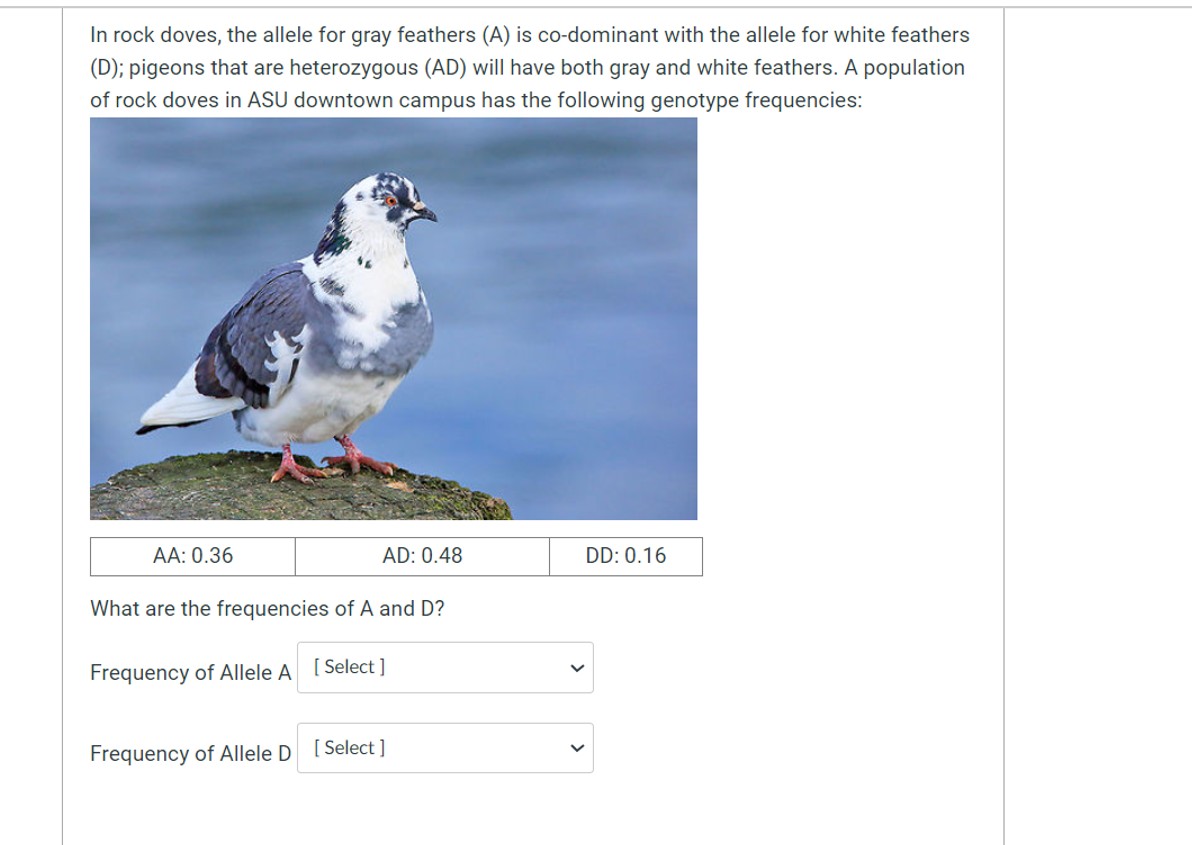This image features a predominantly white background, showcasing a photograph of a medium-sized bird. The bird is characterized by a striking color palette of white, blue-gray feathers, and has distinctive orange feet and a small black beak. It appears to be perched on a wooden post in front of a serene body of water. Above the bird, there is a brief text in gray that reads: "In rock doves, the allele for gray feathers is co-dominant with the allele for white feathers. Pigeons that are heterozygous will have both gray and white feathers. A population of rock doves at the ASU Downtown Campus has the following genotype frequencies."

Beneath this textual information, there are three rectangular boxes displaying genotype frequencies: 
- AA: 0.36
- AD: 0.48
- DD: 0.16

Below these boxes, a question is posed: "What are the frequencies of A and D?" with options to select responses via drop-down menus.